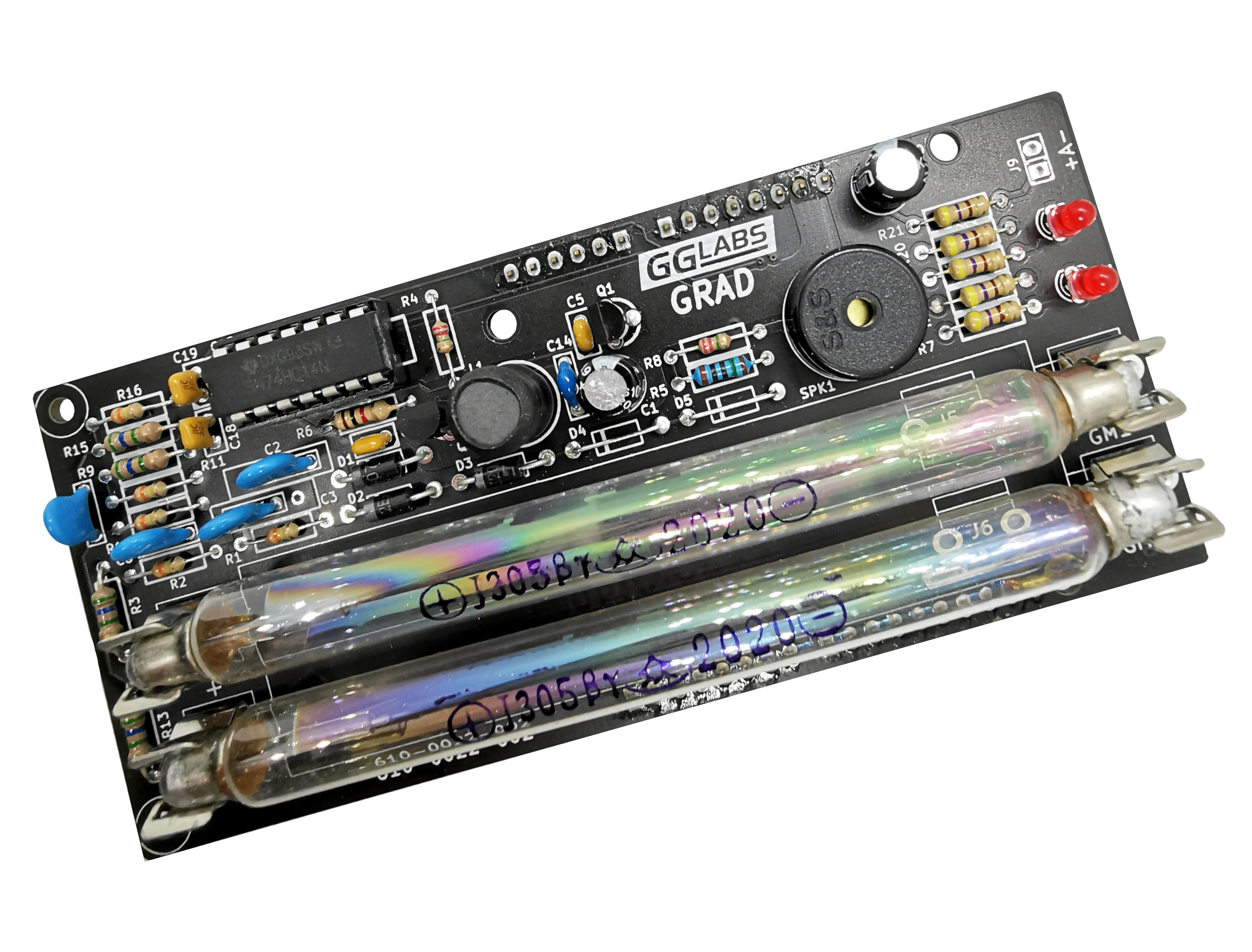The image depicts a close-up shot of a rectangular, black circuit board set against a white background, slightly tilted at a diagonal. The circuit board is densely populated with numerous electronic components, including transistors, wires, and switches of various colors—yellow, red, blue, and more. Notable features include two large, transparent glass tubes running along the bottom half of the board, embossed with the text "J305B2020." Above these tubes are an array of colored switches: two red on the right and five yellow aligned horizontally to their left. Additional switches include those with blue stripes and others combining yellow and red hues. The board also contains different knobs, including one large circular knob labeled "S&S" and a smaller one with a gray interior that lacks text. Tiny boxes, both rectangular and oblong-shaped, are scattered across the top of the circuit board. Markings on the board include random letters and numbers such as "R6," "R21," a plus and minus symbol, and the text "GG Labs, GRAD" along with the "GT Labs" logo, indicating its electronic origin.